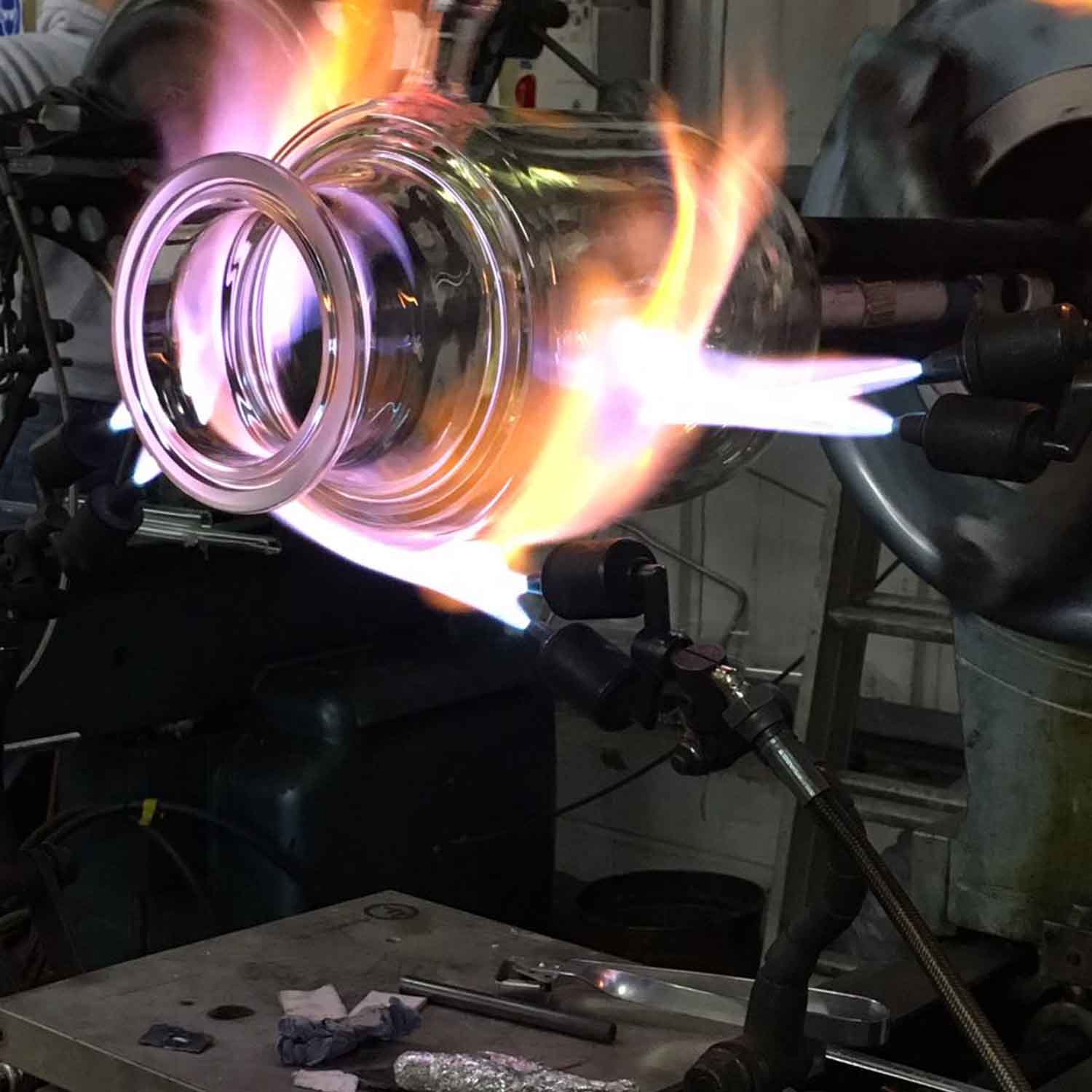The image captures the intricate process of glassblowing in a workshop. At the center of the scene is a clear, cylindrical glass vase being shaped, still connected to a metal rod. The glass is positioned horizontally, reminiscent of an old-style metal milk can. Multiple powerful torches, each with two nozzles, emit a bright blue and violet flame that turns a glowing orange-red upon contact with the glass, indicating the immense heat involved. The torches and the vibrant flames dominate the top two-thirds of the image, creating an intense focal point. Below, the bottom third reveals a metal surface cluttered with various tools and components essential for the glassblowing process. The scene is framed by the metallic structures and connections, including hoses supplying gas to the torches, all indicative of a functional, industrious setting dedicated to the craft of glassmaking.